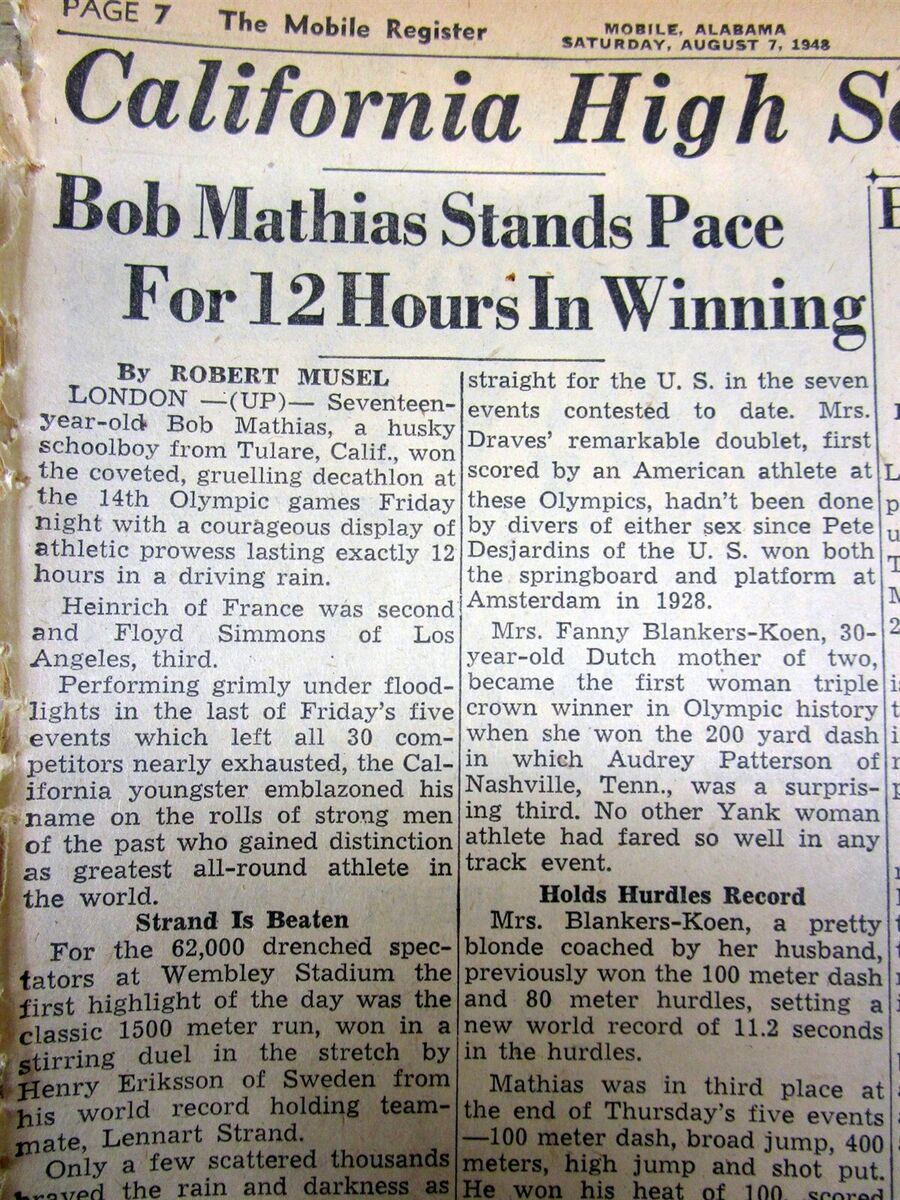This is a detailed photograph of a newspaper clipping from the Mobile Register in Mobile, Alabama, dated Saturday, August 7, 1948, on page 7. The main headline reads "Bob Mathias Stands Pace for 12 Hours in Winning," written by Robert Musel. The article highlights a schoolboy from California, Bob Mathias, who won a grueling decathlon event. The event took place in California and is evidently linked to the 1948 Olympics in London. The narrative includes mentions of other competitors and their performances in the decathlon. Additional sub-headlines within the article state "Strand is Beaten" and "Holds Hurdles Record," with the latter detailing a female athlete described as a "pretty blonde coached by her husband." The upper part of the page is cut off slightly, hinting at "California High S," likely referring to 'California High School.' The clipping is slightly shadowed at the bottom, but the text remains legible.